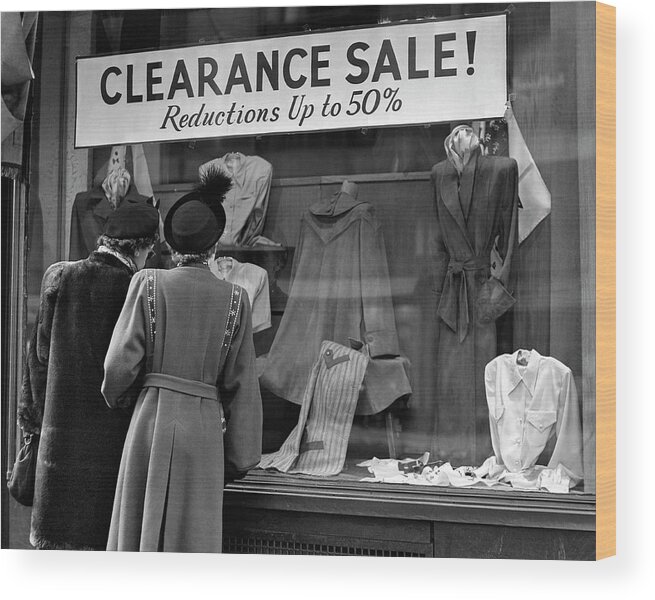This image features a black-and-white photograph that appears to be printed on a canvas set against a white background, giving it a 3D appearance. The canvas is not framed but seems designed to be hung up. In the photograph, two women, dressed in 1940s fashion with long coats and fancy hats, are gazing into a storefront window display. Above the store window, a sign reads "Clearance Sale: Reductions Up to 50%." The window display features various articles of clothing, including a skirt, coat, dress, and a white shirt at the bottom. The lack of color, with shades ranging from light to dark gray, emphasizes the vintage feel of this scene.